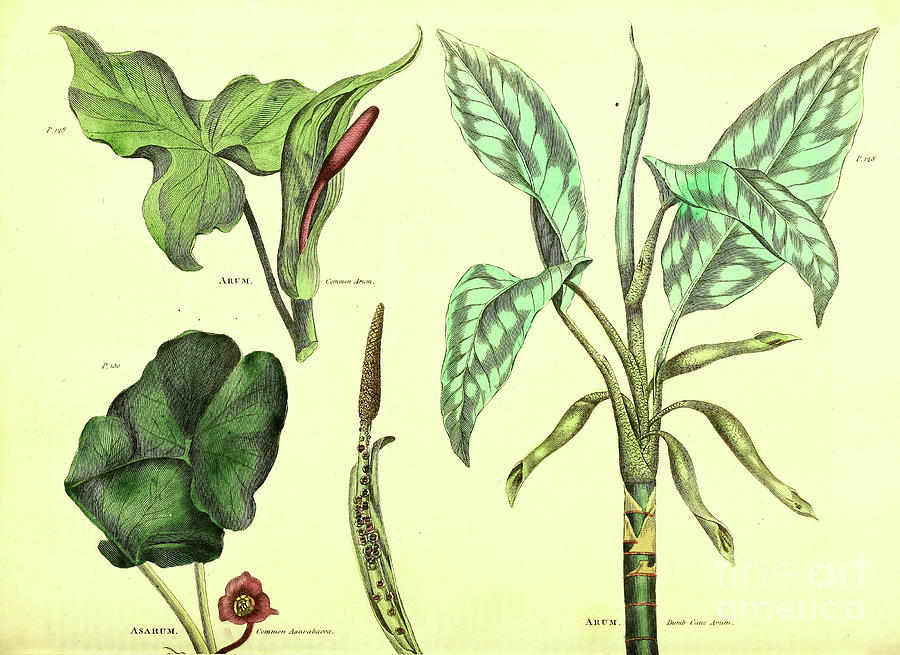This image, seemingly from a plant identification book, showcases detailed illustrations of four distinct plants. In the top left corner, there's a depiction of a common arum, characterized by a green leaf branching into three parts and a pinkish, nodule-like structure on the stem. Below it is another plant, resembling a clover with a prominent red flower. The central illustration features a simplistic design of a single stem with no accompanying leaves. To the right, the image displays a dumb cane plant, notable for its bamboo-like stem and large, distinctively marked green leaves. The text accompanying these illustrations is very small and difficult to read, but the intricate details and styles of the drawings are typical of field guides used for plant identification.